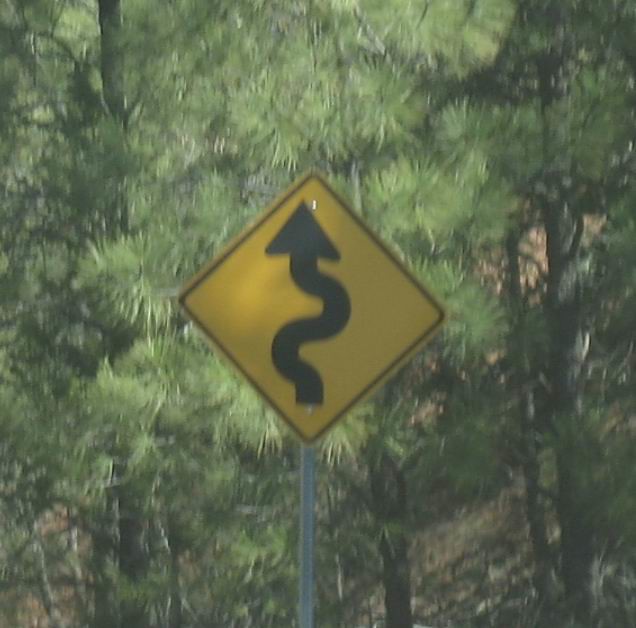The photograph captures a roadside warning sign prominently displayed against a lush, green forest backdrop. The vibrant yellow sign, which is triangular in shape and outlined in black, features a black squiggly arrow starting straight at the bottom, curving left and right, then straightening out before reaching the top. This sign is securely attached to a light gray, narrow rectangular metal post with two bolts. The background consists of a dense forest with both dark brown and gray tree stumps at the bottom and a mix of light and dark green leaves higher up. The entire scene is bathed in daylight, clearly indicating to motorists that a curvy road lies ahead.